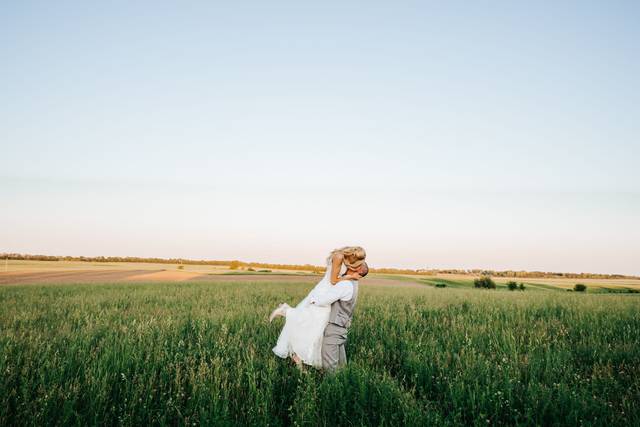The image captures a romantic moment between a couple sharing a kiss in what seems to be a wedding photograph. The woman, with long blonde hair, is wearing a long white dress that resembles a wedding gown and white shoes. The man, possibly with gray hair, is dressed in light gray dress pants and vest over a white shirt. He lifts her off the ground while they kiss, her feet slightly elevated. They are standing in the middle of a field with tall, green plants reaching up to knee height. Behind them, an expansive landscape stretches out, featuring fields in varying shades of green and light brown, dotted with patches of trees. Above them, a clear, light blue sky completes the picturesque scene.